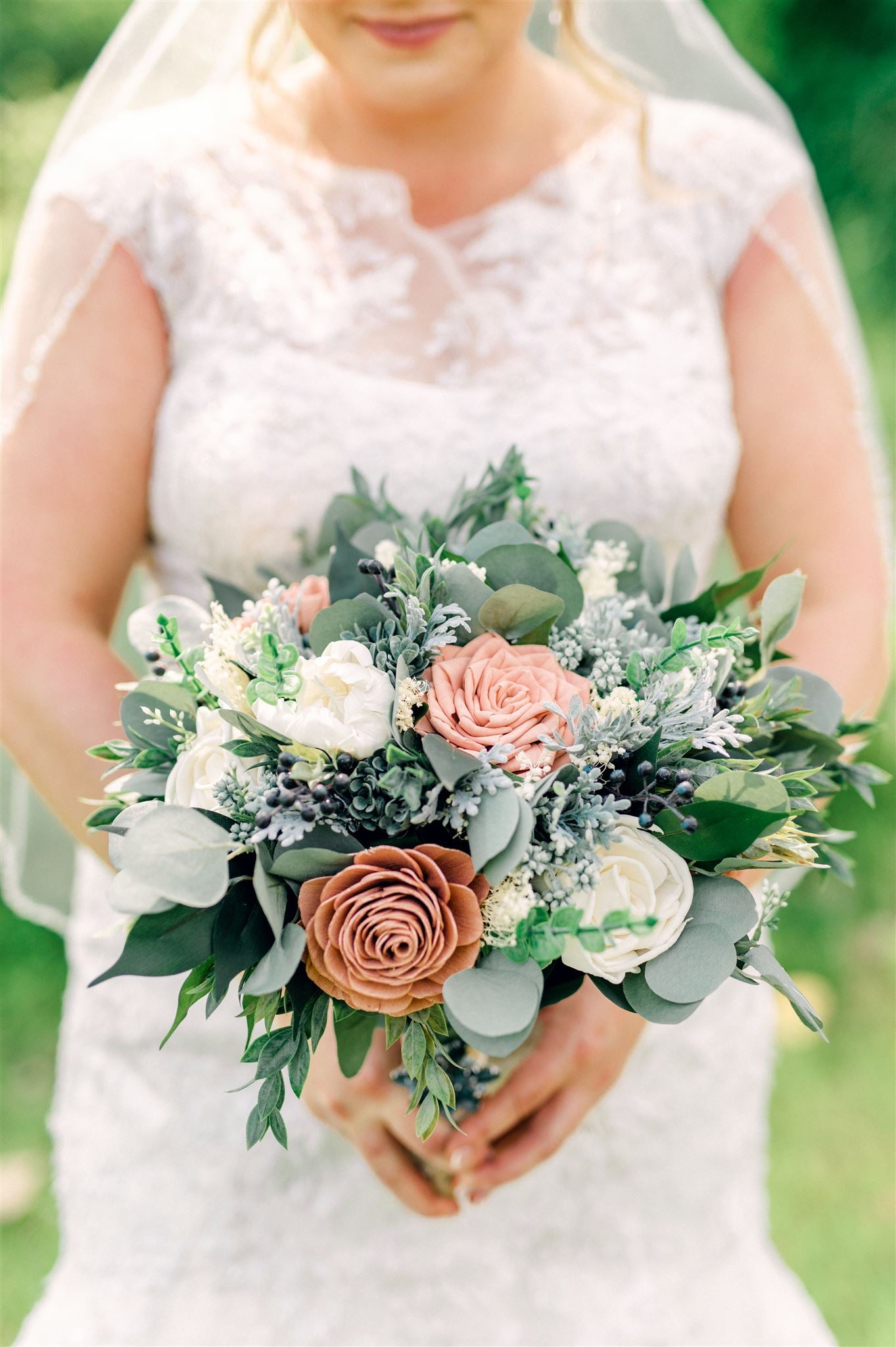A color photograph in portrait orientation depicts a bride holding a bouquet of flowers. The bride, who has long blonde hair cascading in curls and is smiling, is captured from just above her nose to just below her hips. She wears a white bridal gown with short sleeves and a clear white veil. The focus of the image is on the bouquet she holds with both hands in front of her hips. The bouquet features a variety of flowers, including white roses, orangish-pink roses, and assorted greenery, possibly eucalyptus leaves. The flowers’ colors range from dark russet to light peach and white, giving them a vintage appearance. The background is slightly out of focus, emphasizing the bouquet and giving a dreamy quality to the bride, who fades softly into the green backdrop.